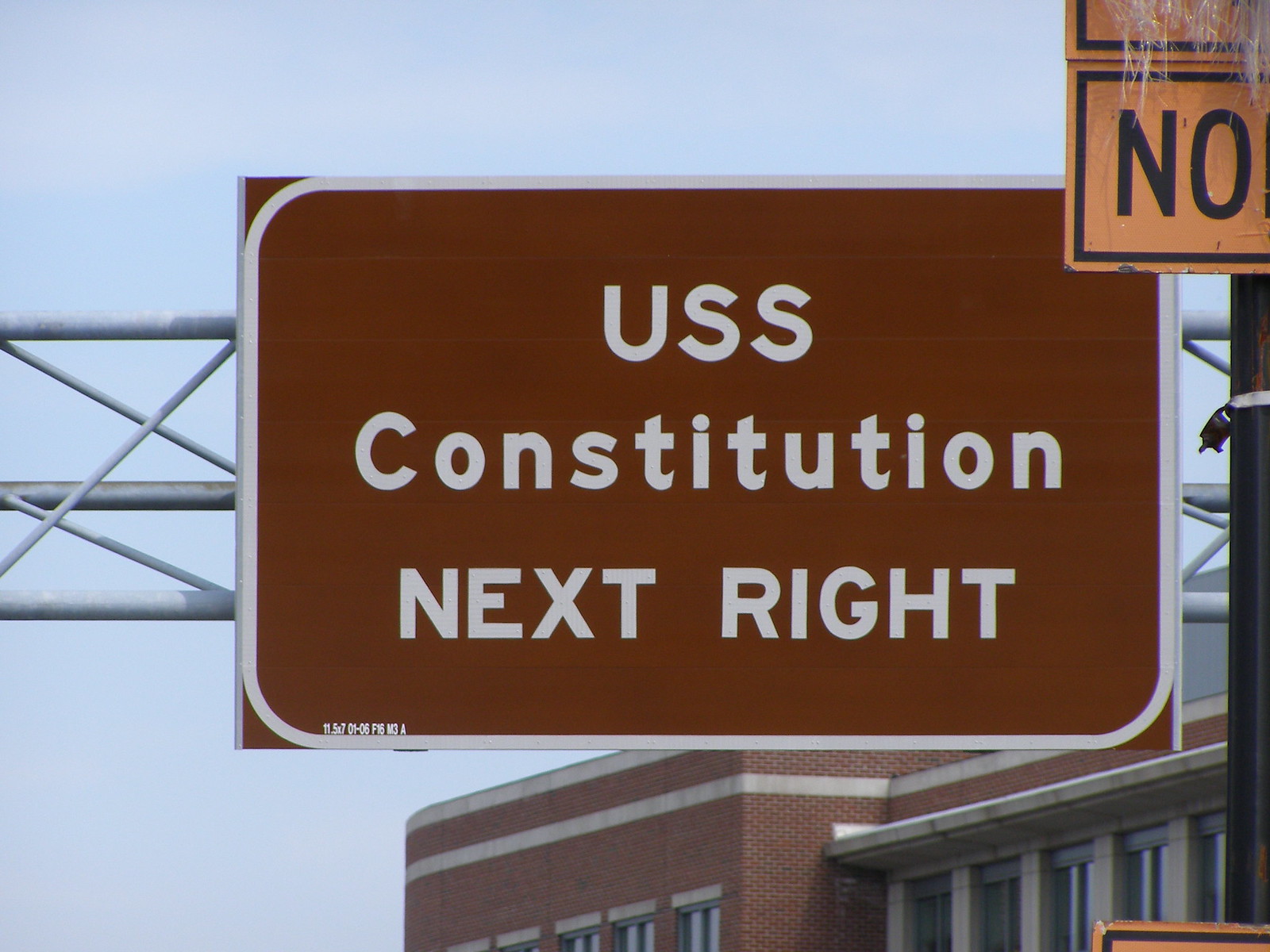The photograph captures a detailed, close-up view of an outdoor highway sign. The primary focus is a brown sign with white text that reads "USS Constitution" with an arrow indicating the "NEXT RIGHT." The sign is mounted on a sturdy metal bracket designed to extend over the road. In the upper right corner, an amber sign with black text partially visible, displaying a large "NO," implying a no-parking regulation.

In the background, almost dominating the foreground due to the zoomed-in perspective, stands a brick building. The façade is primarily red brick with off-white brick trim. The architectural details include a light-colored horizontal border of bricks near the roofline, and a section of the building is recessed, featuring additional windows and an overhang. This suggests that the structure may be a large, official building. The scene is devoid of other elements, focusing solely on the signage and the architectural detail.